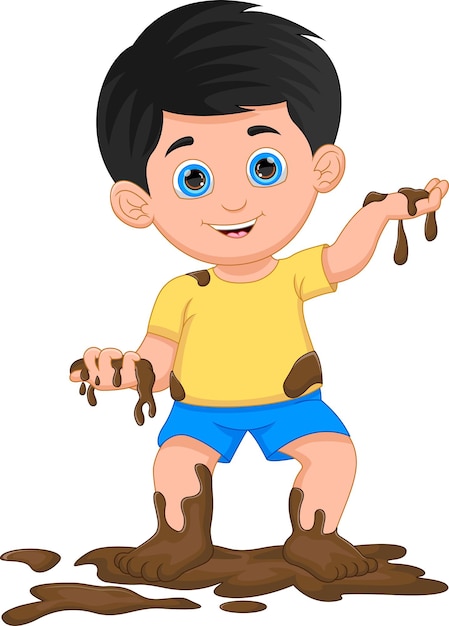This detailed color illustration, likely a drawing or painting, shows a young boy of about three years old standing joyfully in a muddy substance, possibly melted chocolate. The image is in portrait orientation, and the background is white, drawing all focus to the child. He has round blue eyes, peach-colored skin, and black hair neatly combed to the side. The boy is wearing a light yellow (gold) t-shirt and blue shorts, both of which have brown splotches of the mysterious liquid. He is depicted with a smile, facing the viewer, and his arms are raised beside him. One hand, held up beside his face on the right side of the image, has the brown liquid dripping from it, while the other hand on the left side has fingers curled backward, also holding the brown substance. His legs are similarly smeared, with the liquid dribbling down his calves and ankles, pooling irregularly around his feet. The artist has meticulously captured the boy's playful engagement with the mud, emphasizing the fine details like the mud falling through his fingertips and the striking shade of his light blue eyes.